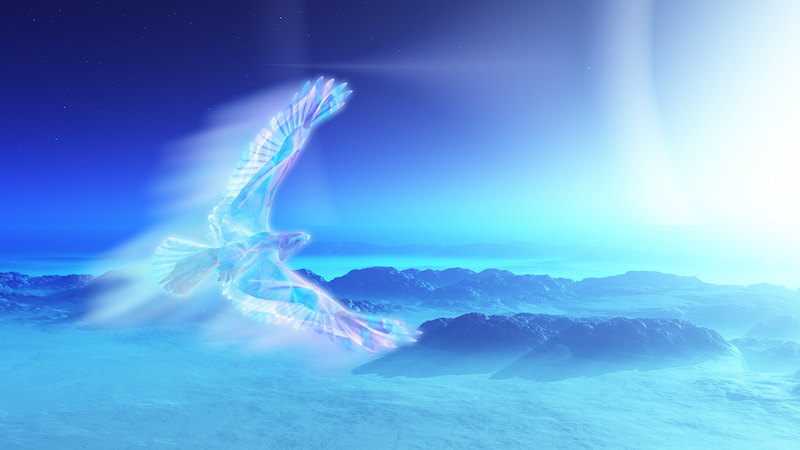This is a rectangular, computer-generated image likely set in a fantastical Arctic-like landscape. Dominated by cool tones of blue, purple, and teal, the image showcases a surreal environment. The snowy terrain below is highlighted with aqua blue hues, contrasting against dark gray-blue rocky cliffs and mountain ranges that stretch towards the horizon. In the distance, a mystical fog, blending shades of green-blue and white, drifts through the scene, enhancing the ethereal atmosphere.

Above this alien terrain, a crystalline bird soars majestically from the left, its translucent wings outstretched. The wings, significantly larger than its small body, sparkle with a spectrum of colors including whites, blues, purples, and hints of pink, reflecting the light that streams through. A trailing blue light follows the bird, adding a dynamic sense of motion.

The sky overhead is a gradient of unreal blues, darker on the left and transitioning to a lighter shade towards the right. Pinpoints of white stars twinkle against this celestial backdrop, and an aurora-like effect dances on the right side, alongside a radiant white light that could suggest a fantastical sunrise or otherworldly phenomenon. This detailed and vivid scene suggests an imaginative rendition of an Arctic landscape, brought to life with meticulous digital artistry.